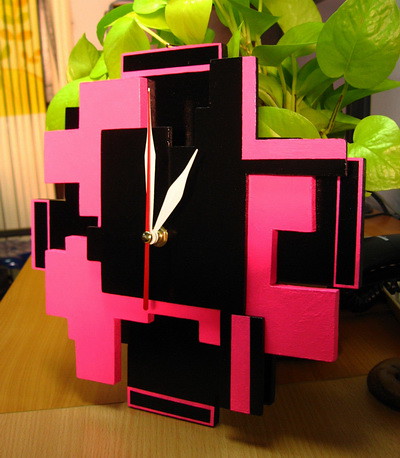This image showcases a strikingly contemporary clock, characterized by its geometric design composed of various overlapping shapes that lend depth and dimension. The clock employs a bold palette of hot pink, transitioning through a spectrum from orangey-pink to lighter pink, juxtaposed against black elements. Its form is loosely square, with one of its corners extending upward into a neighboring area, adding an avant-garde touch. 

The clock's face features minimalist white hands with pointed ends, showing the time as either one o'clock or two o'clock, complemented by a prominent red second hand pointing directly at where the 12 would be positioned, though the clock lacks numerical markers. 

Behind the clock is a backdrop of heart-shaped leaves from a nearby plant, adding an organic contrast to the clock's modern aesthetic. The scene is set on a brown desk, with a hint of cream and tan drapes in the background. The desk holds other indistinct items, partially obscured and cast in shadow, indicating the presence of light shining down from above, enhancing the overall depth and mood of the composition.